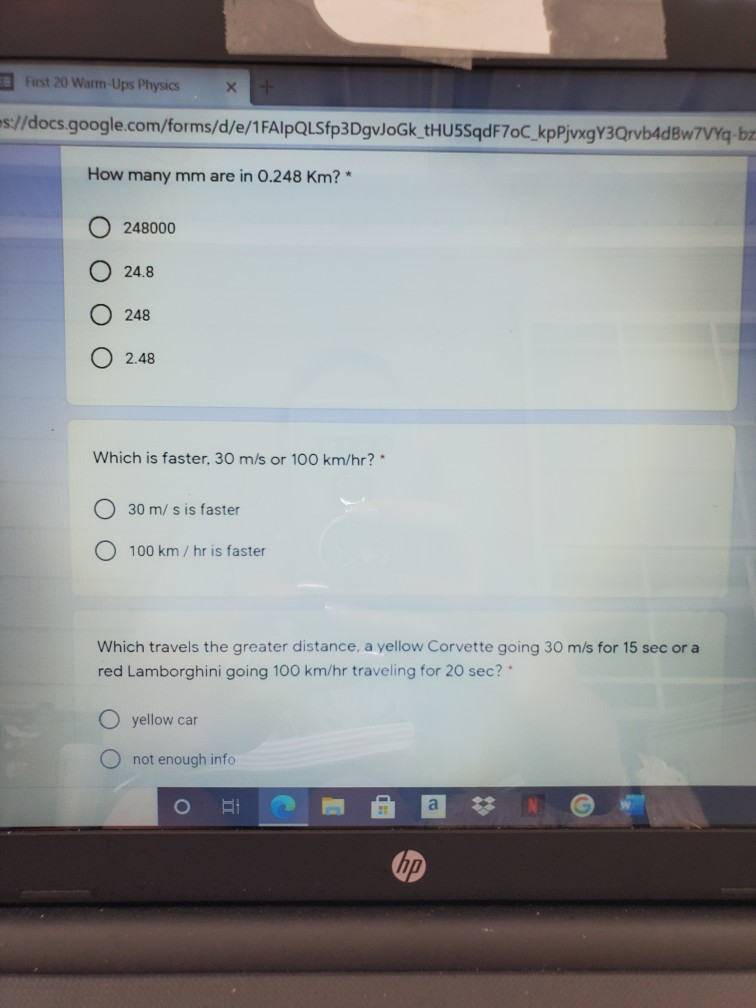In this image, we see a person, appearing to be white-skinned, holding a camera with both hands, capturing a photo of their computer monitor. The monitor displays a web browser with a single tab open, titled "First 20 Warm Up Physics." The URL in the address bar begins with "docs.google.com/forms/d/eth" followed by a lengthy string of letters and numbers.

The main content on the screen is part of an online physics quiz. The first visible question asks, "How many mm are in 0.248 km?" The multiple-choice answers provided are:
1. 24800
2. 24.8
3. 2.48
4. 248000

Below that, another question reads, "Which is faster, 30 m/s or 100 km/h?" with two possible answers:
1. 30 m/s is faster
2. 100 km/h is faster

The final section shown presents the question, "Which travels a greater distance, a yellow Corvette going 30 m/s for 15 seconds or a red Lamborghini traveling 100 km/h for 20 seconds?" The answer choices are:
1. Yellow car
2. Red car
3. Not enough info

The detailed elements of this image, from the individual taking the photo to the specifics of the quiz questions, capture a moment focused on studying or preparing for a physics assessment.